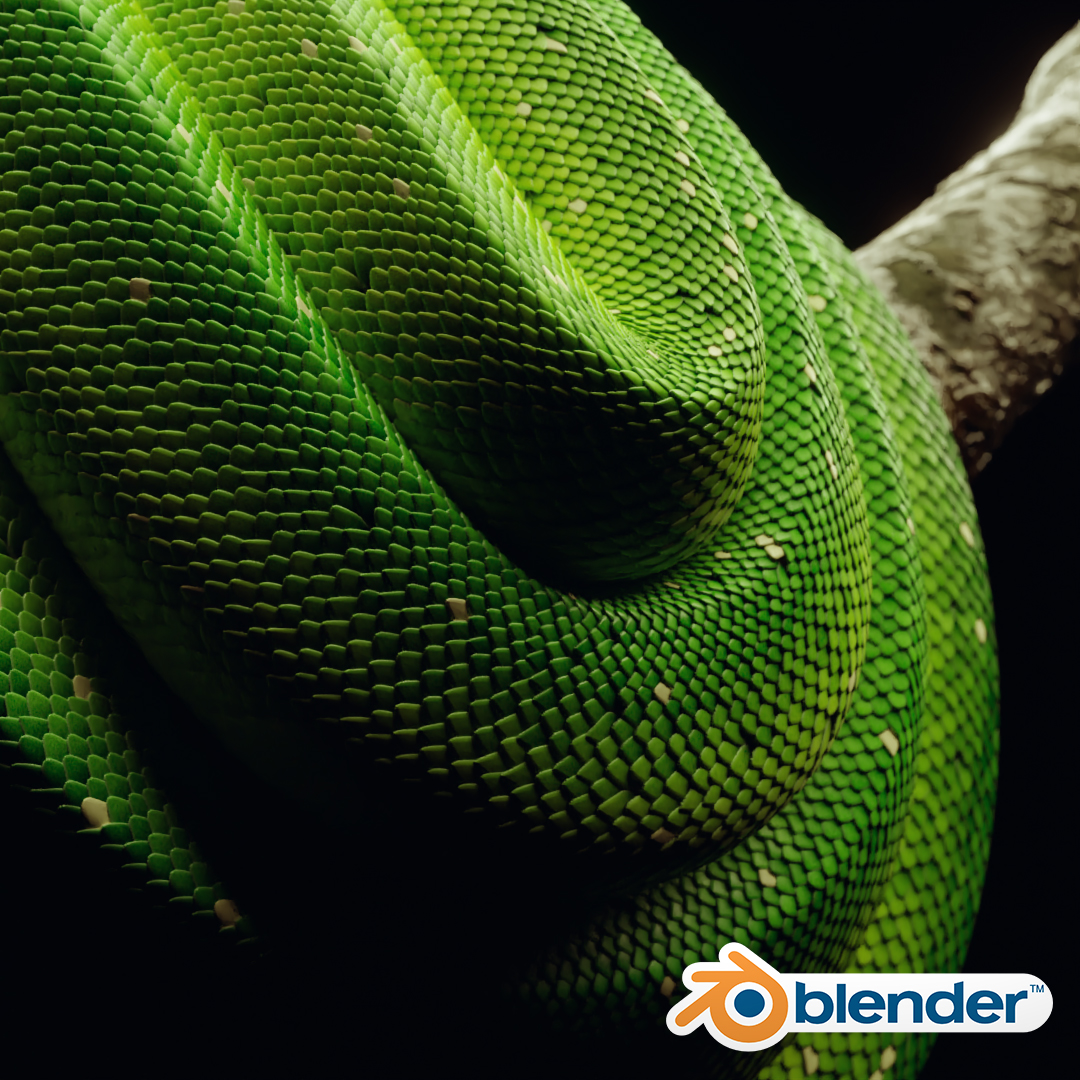The image depicts a strikingly green python coiled up on a rough, grayish-brown tree branch that extends to the upper-right corner against a black backdrop. The snake's vibrant, perfectly aligned scales, interspersed with subtle hints of white, create a striking visual contrast with the branch. However, neither the python's head nor tail is visible, adding an element of mystery to the scene, which some might speculate looks almost too perfect, almost artificial. In the lower part of the square-shaped photo, there is a distinctive logo featuring the word "Blender" in blue letters with a small trademark symbol. To the left of the text is an emblem: an orange circle with a blue dot in the center and orange points extending to the left.